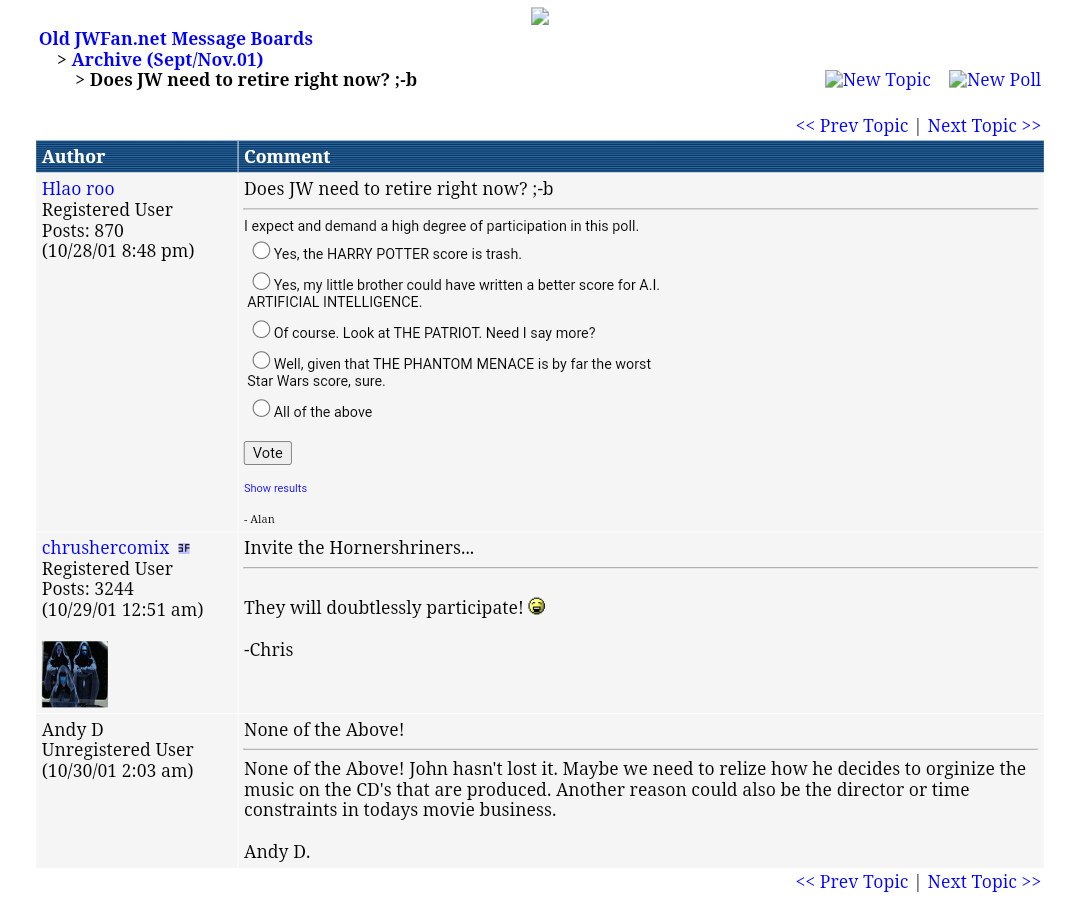A group of individuals are seen collaborating intensely around a state-of-the-art trailer, meticulously discussing and selecting various equipment and gear for an upcoming event. The setting is bustling with activity as Harry Potter scores play in the background, adding an air of whimsical enthusiasm to the scene. Lively debates ensue over the musical arrangements and orchestration choices, with some humorously noting that even a little brother could contribute to the compositions. Additionally, a variety of comic and patronage memorabilia are scattered around, indicating a passionate dedication to the thematic elements of the event. Amidst the vibrant discussion, there is also an evident camaraderie and shared excitement about the involvement of horse riders and their expected enthusiastic participation. The scene vividly captures the essence of collaborative creativity and the organizational prowess required to pull off such an elaborate event, all while balancing humor, dedication, and a shared love for the arts and community.